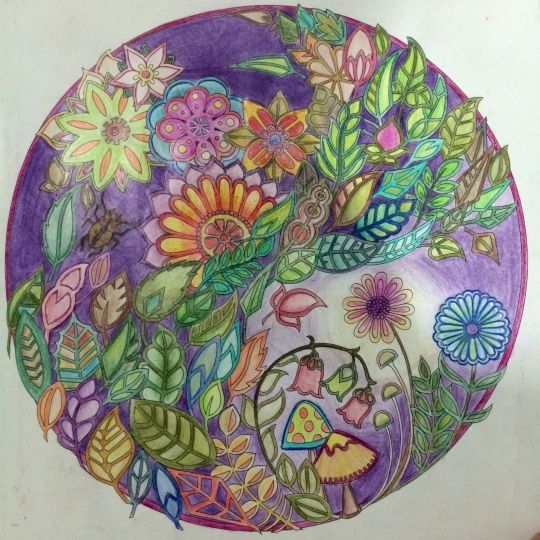The image is a hand-drawn, colourful illustration captured in a square photograph. This intricate drawing is enclosed within a thin, mauve circumferential line. Extending beyond this boundary, particularly between the 9 o'clock and 6 o'clock position in the bottom left, are illustrated leaves that add a sense of liveliness to the composition. The illustration is an imaginative and vibrant interpretation of nature, with a multitude of colours and elements crammed within the circular frame.

Dominating the interior space are various colourful leaves drawn in unconventional hues such as yellow, blue, mauve, and orange. These leaves are interwoven with each other in some places, creating a collage-like effect, while in other areas, they are set against a plain purple background created with coloured pencils. Scattered among the foliage are a number of flowers, depicted in an array of colours: red, yellow, green, blue, pink, and purple, each vividly contrasting with the others.

Complementing the floral diversity are small mushrooms and toadstools, detailed in unique colour combinations like blue bodies with green tops and red spots, or yellow bodies with dark red outlines. Tiny butterflies and a small brown beetle add more life to the scene. The background itself transitions from darker purples at the top to lighter purples at the bottom, enhancing the depth and beauty of this nature-inspired art piece. Overall, this artistic creation is a joyful and detailed exploration of nature, captured within a striking purple-bordered circle.